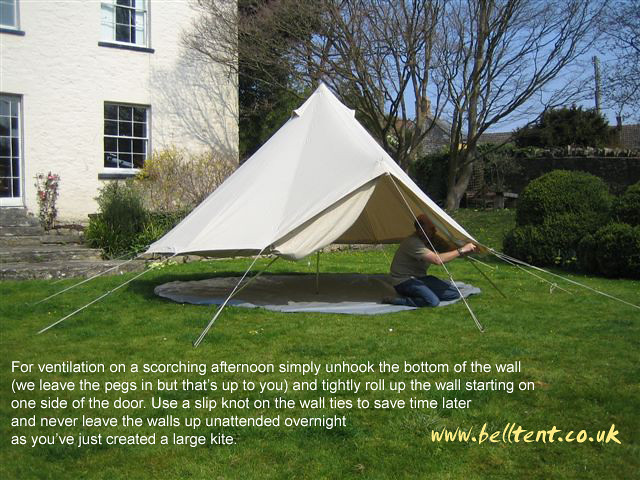The photograph, taken outdoors on a clear, sunny day with a blue sky, captures a lush, green grassy yard in front of a beige or off-white cream-colored house. The house is partially visible, showing a few windows and concrete steps leading into it. In the center of the image, a middle-aged, balding man, dressed in a beige short-sleeved shirt and blue jeans, is kneeling and adjusting the final tie-outs of an off-white, creamy beige circular tent. The tent, which is partially elevated about two feet off the ground, features multiple tie-outs and stakes. Behind the man, there are some green shrubs and leafless trees, with another house visible in the background. At the bottom of the image, text from the BelTent website (www.beltent.co.uk) promotes the tent describing features like ventilation advice and usage instructions, emphasizing the convenience of unhooking the bottom of the tent walls for better airflow.